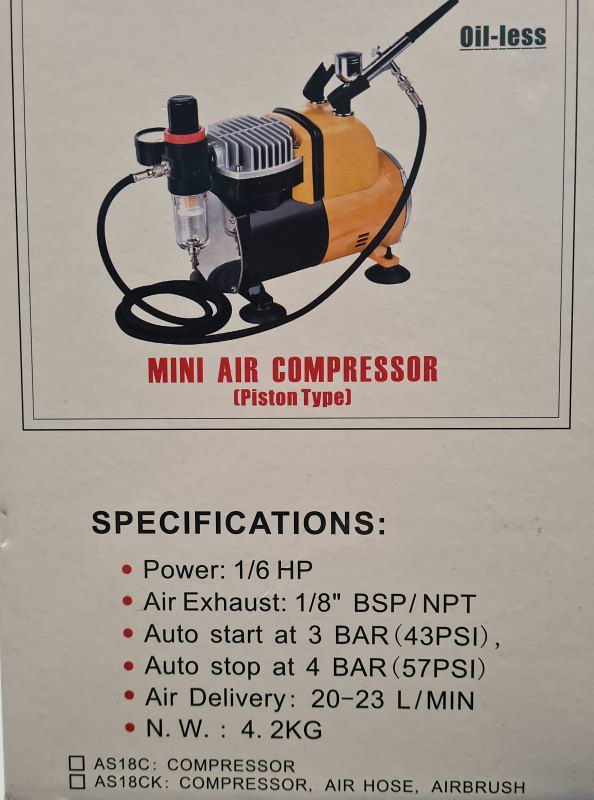The image depicts a single, slightly aged white poster that takes up the entire frame. At the top, there is a black and yellow mini air compressor with an attached airbrush via a rubber hose. To the top right, bold text reads "Oil-less," followed by "mini air compressor, piston type" beneath it in red with parentheses. The specifications listed in black text below include: power 1.6 HP, air exhaust 1/8 BSP/NPT, auto start at 3 bar (43 PSI), auto stop at 4 bar (57 PSI), air delivery of 20-23 L/min, and a net weight (NW) of 4.2 KG. The poster's background colors include tan, black, yellow, red, gray, and silver. A mention of potential purchase options includes "compressor" and "compressor, air hose, airbrush." The overall look suggests that this is a product sheet for a tool on sale, reinforced by a boxed area with a check mark, indicating order options.